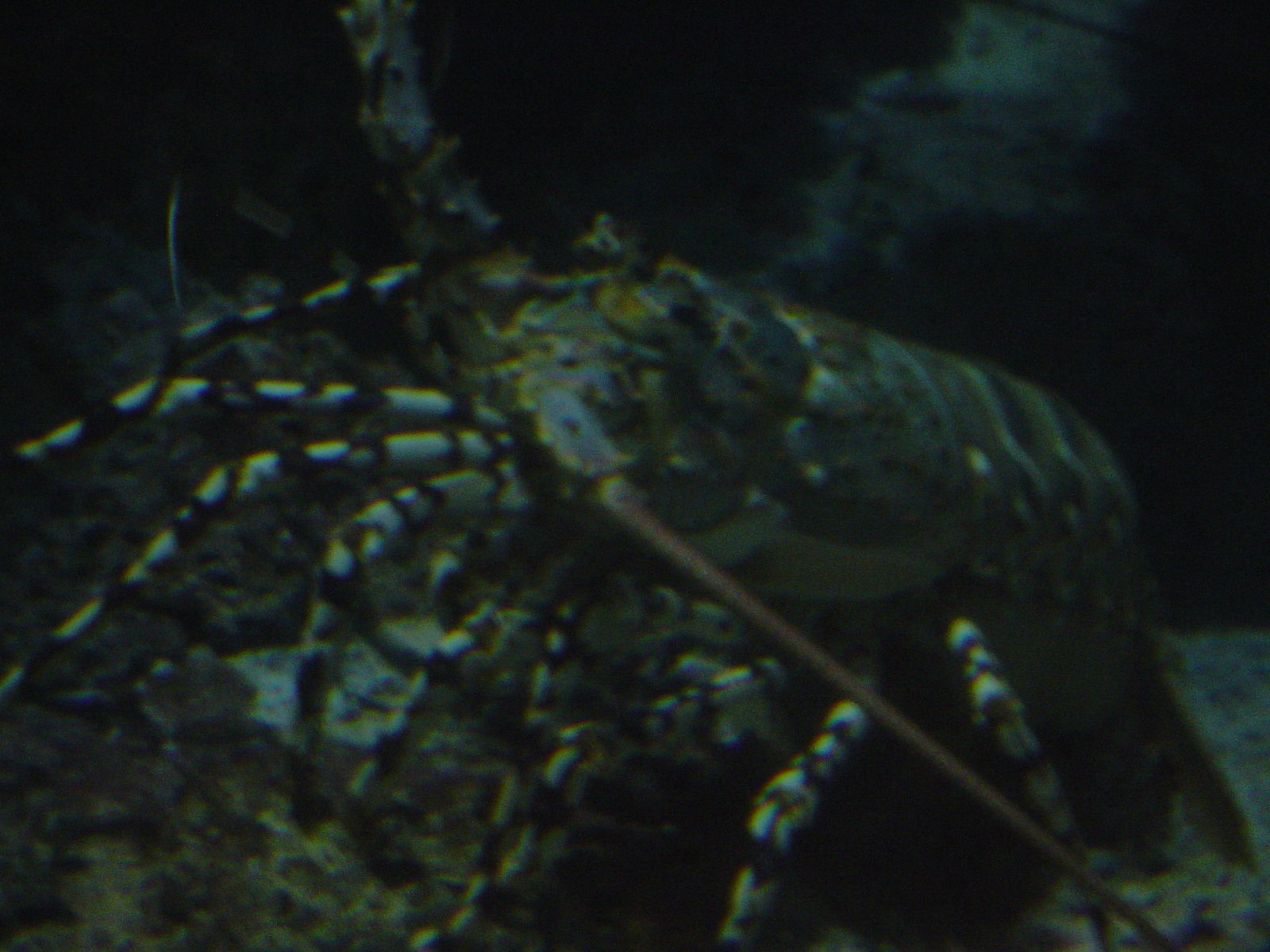This underwater close-up image captures a single lobster intricately sprawled over a mottled, large rock. Dominating the center to the right, the rock's dark hues blend seamlessly with the ocean's deep blue-black backdrop, giving the scene a moody and mysterious ambiance. The lobster's many legs, vividly striped with white and blue, fan out prominently in front of its armored body as it seemingly moves from the lower right to the upper left. Its body exhibits a striking palette of blue, black, and hints of green, matching the rocky surface it navigates. Long antennae project from the sides of its head, extending towards the bottom right of the photo. The lobster's detailed texture, along with the dark and somewhat blurry environment, suggest the photo was taken underwater, possibly in a natural ocean setting or a large aquarium.